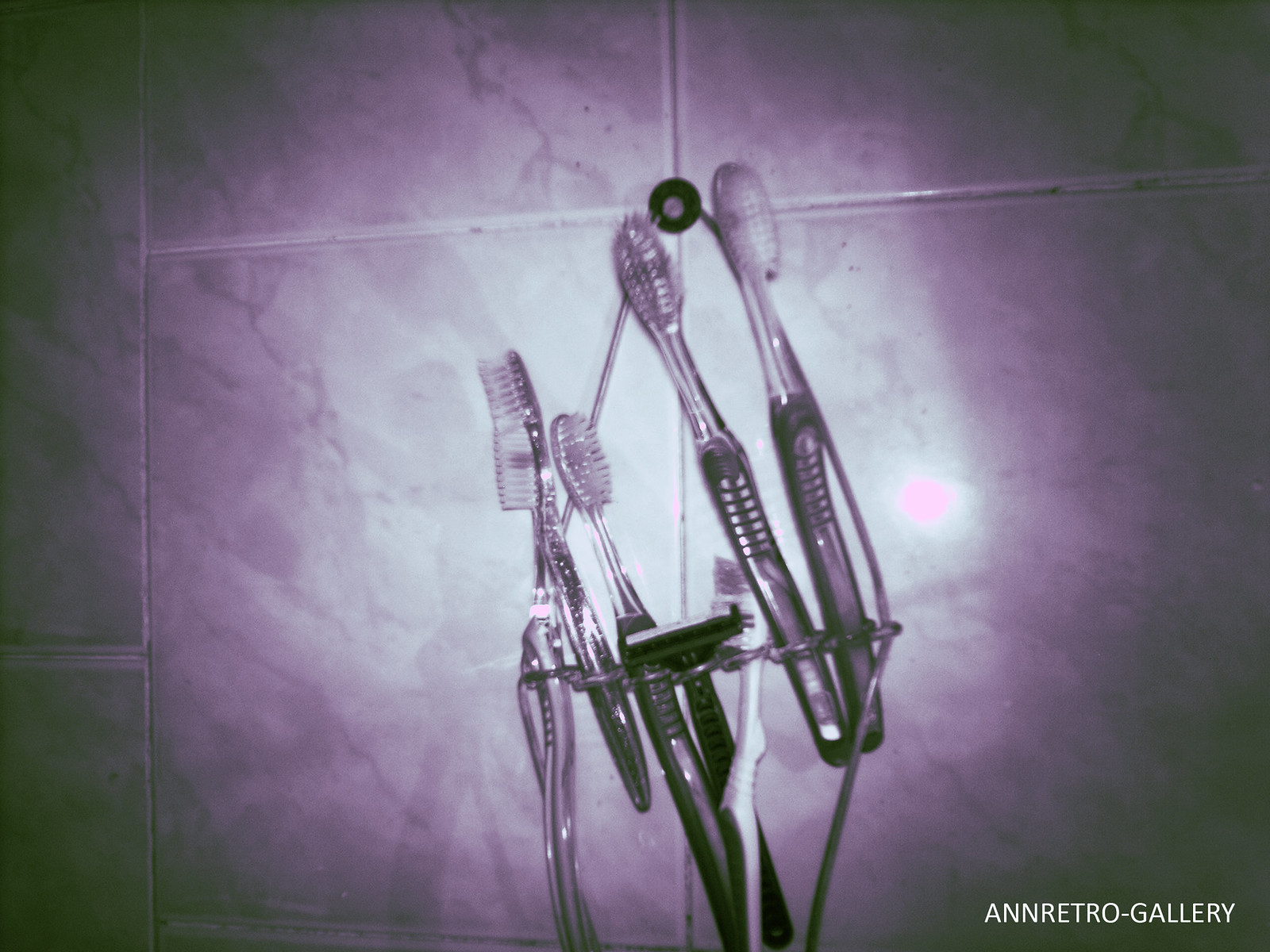The black and white photograph depicts a toothbrush holder mounted on a marbled tile wall typical of a bathroom setting. The metal holder, fastened to the wall with a black loop at the top of its wire structure, contains six toothbrushes and a disposable razor. The holder's wire frame includes vertical and horizontal components with loops to slot various objects. Among the toothbrushes, most have wide handles and sit directly above the loops, while one toothbrush with a finer handle has fallen and rests on its head. The disposable razor is positioned with its blade resting on the end of the rack. A strong light source, likely from a camera flash, illuminates the toothbrushes, casting a flare. The background tiles appear light-colored due to the grayscale image, with a potential light purple reflection. The bottom right corner of the image includes the text "A-N-N-R-E-T-R-O/G-A-L-L-E-R-Y," while the photo itself has darker gray corners, with the center brightly lit.